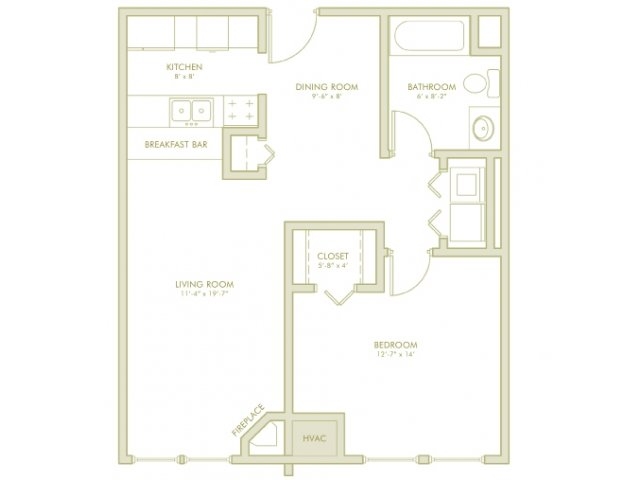The floor plan illustrates a house or apartment layout with distinct rooms and features. In the bottom left corner, there is a spacious living room, which is accessible through two doors on its front side. A unique triangular-shaped fireplace is situated towards the bottom right of the living room. The kitchen, measuring 8x8, occupies the top area of the plan and contains essential appliances, including a sink and what appears to be either a stove or a dishwasher, integrated into the countertop. Below the kitchen, a breakfast bar offers a convenient dining space. Adjacent to the kitchen on the right, there is an open dining room highlighted by a semi-circular bay extending from the wall, adding an elegant touch. Moving further to the right, a bathroom is positioned for easy access, and directly below it, a cozy bedroom features a built-in closet for ample storage.